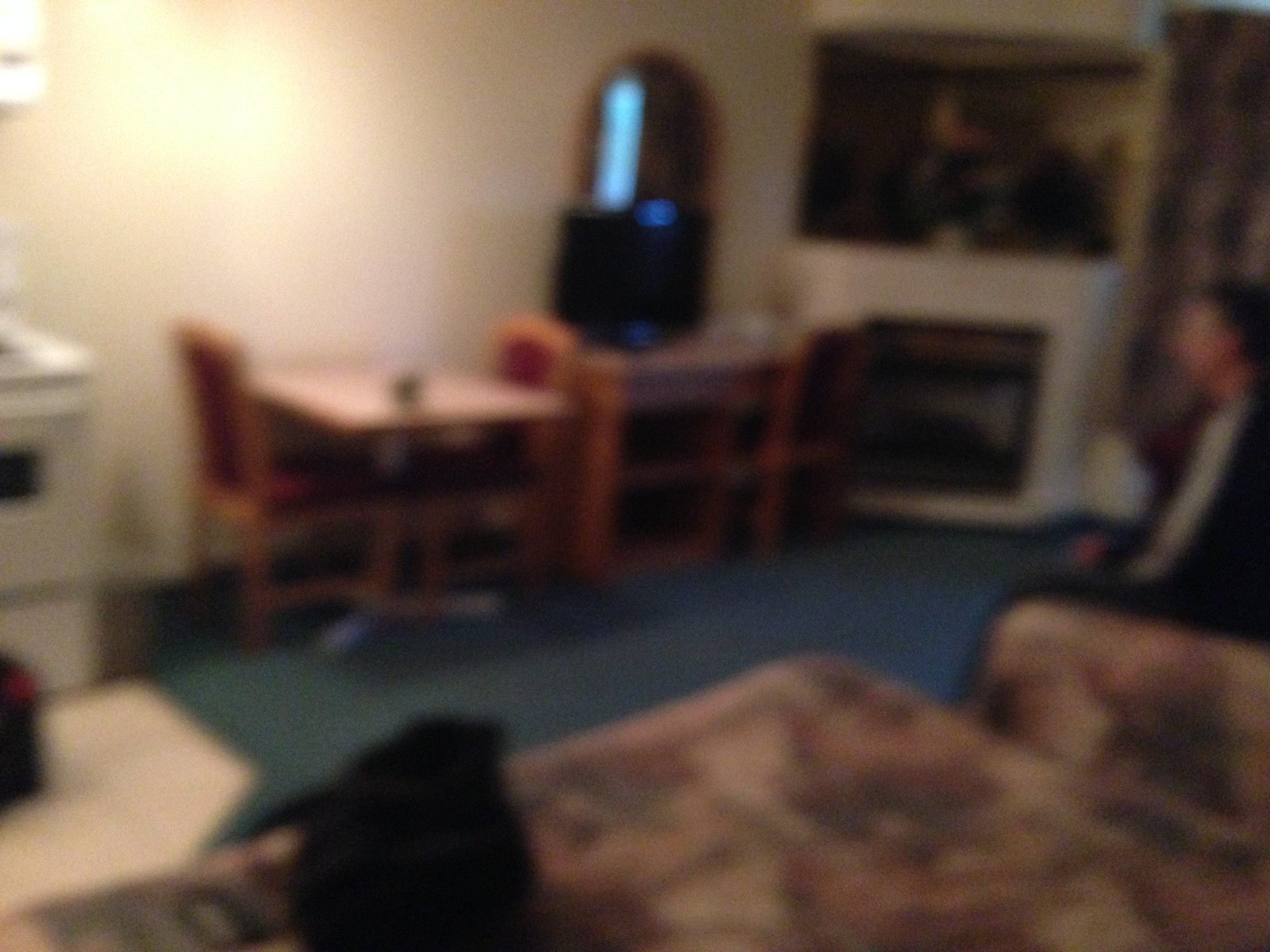This photograph captures the blurry and grainy interior of a home, making it difficult to discern fine details but still allowing visibility of basic shapes and outlines. In the background, a white wall sets the stage for a modestly furnished room. Against this wall stands a small table accompanied by two chairs, one on each side. The table features a central object, perhaps a decorative piece, with colors appearing to range from darkish to light brown. The chairs are likely yellow in color. Covering the entire room is a blue carpet.

To the right of the table, a vanity or dresser with a large mirror is visible, with what appears to be a computer screen or smaller TV positioned in front of it. Further to the right, the corner of the room houses what seems to be a fireplace, although it is too dark to see what is on top of it clearly. Below, a square shape close to the ground confirms the presence of the fireplace.

On the extreme right edge of the image, a person is partially visible, sitting on what could be a sofa or recliner adorned with a floral pattern. The person appears to be a white male with short hair, wearing dark clothing with a white stripe. The view offers only the left side of him.

The bottom of the image also features the floral pattern, likely from the mentioned furniture. To the left side of the photo, an appliance suggests that the room connects to a kitchen. The appliance, looking like a white stove, hints at the culinary area adjacent to the living space.